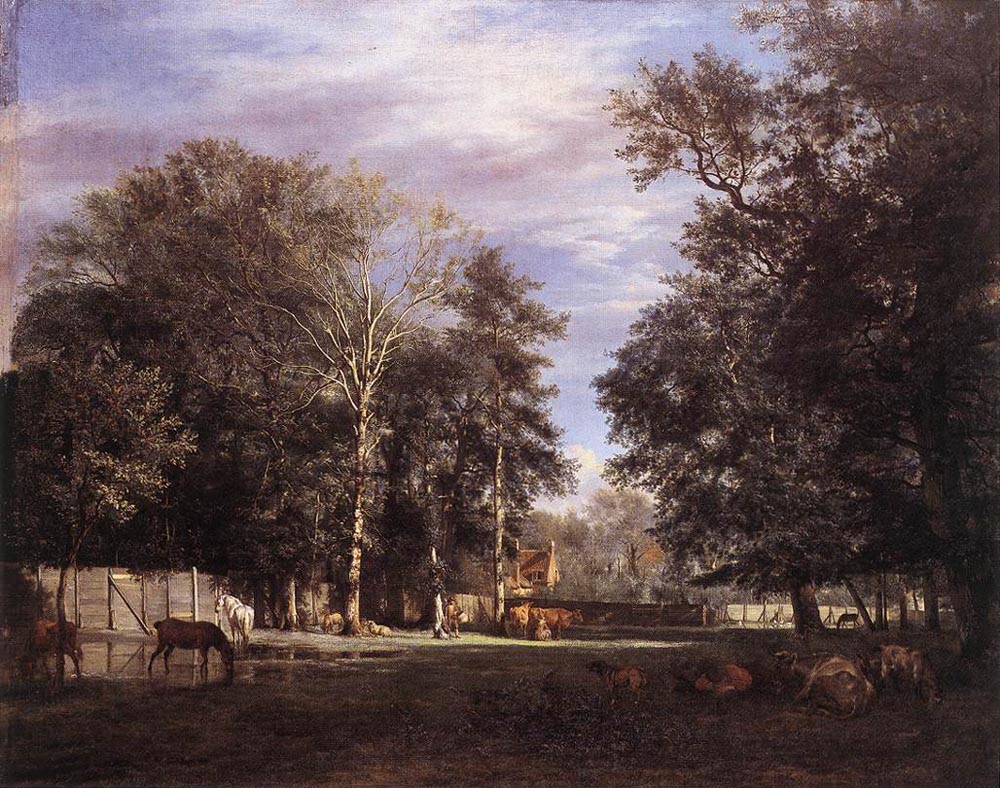The image captures an exquisitely detailed and realistic oil painting of a tranquil European farm scene. Dominating the landscape are large deciduous trees, some with dark brownish bark and green leaves, framing the scene on either side. Towards the middle left stands a particularly bare tree with lighter bark. The vibrant blue sky overhead features wispy white clouds, casting a serene light on the landscape beneath. 

In the foreground, a lush, grassy expanse is populated by various farm animals. Horses of different colors, including brown and white, are seen grazing and standing near patches of standing water. Cows recline in the shade, and dogs can be seen resting towards the bottom right of the image. A small figure, possibly a child, kneels beside a tree, adding a tender human element to the pastoral setting.

A sturdy wooden fence runs along the left side and extends into the background, where another fence partially bisects the scene. Further in the distance, nestled among the trees, stands a charming European-style house with beige-reddish walls and a reddish roof. The lighting in the painting reveals both shaded areas in the foreground and sunlit regions deeper into the scene, emphasizing the depth and realism of the artwork. The overall ambiance is one of serene rural life, beautifully captured in meticulous detail.